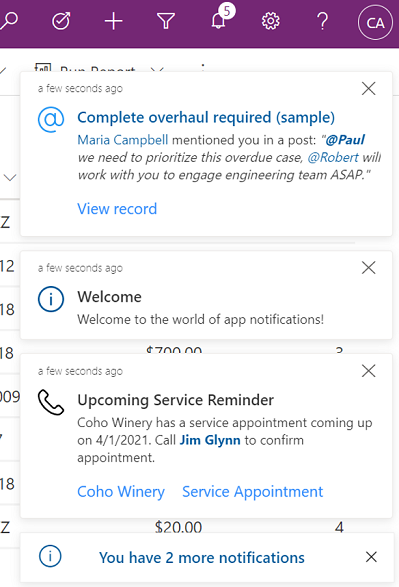This is a detailed screenshot of a phone interface with various notifications and options displayed. 

At the top, there is a dark purple banner featuring several icons from left to right: a search symbol, a check mark, a plus sign, a funnel, a bell with the number five on it, a settings gear, a question mark, and the initials "CA" enclosed in a circle. 

Below this banner, there are four rectangular notification boxes:
1. The first box, marked as "a few seconds ago" in pale gray lettering, includes an '@' symbol followed by the message: "Complete overhaul required sample. Maria Campbell mentioned you in a post: 'Paul, we need to prioritize this overdue case ASAP at Robert. We'll work with you to engage the engineering team ASAP.'" A clickable "View Record" link is provided beneath this text.
2. The second box, also timestamped as "a few seconds ago," displays an 'i' in a circle next to a welcoming message: "Welcome to the world of app notifications."
3. The third rectangle, indicated with "a few seconds ago" and featuring an image of a phone handset, reads: "Remaining service reminder: Coho Winery has a service appointment coming up on 4-1-2021. Call Jim Glenn to confirm the appointment." The names "Jim Glenn," "Coho Winery," and the term "service appointment" are highlighted in blue font.
4. The final notification box presents an 'i' in a circle with the text: "You have two more notifications," highlighted in blue.

Each notification provides quick insight into recent activity and reminders, offering interactive elements like clickable text and links for user engagement.